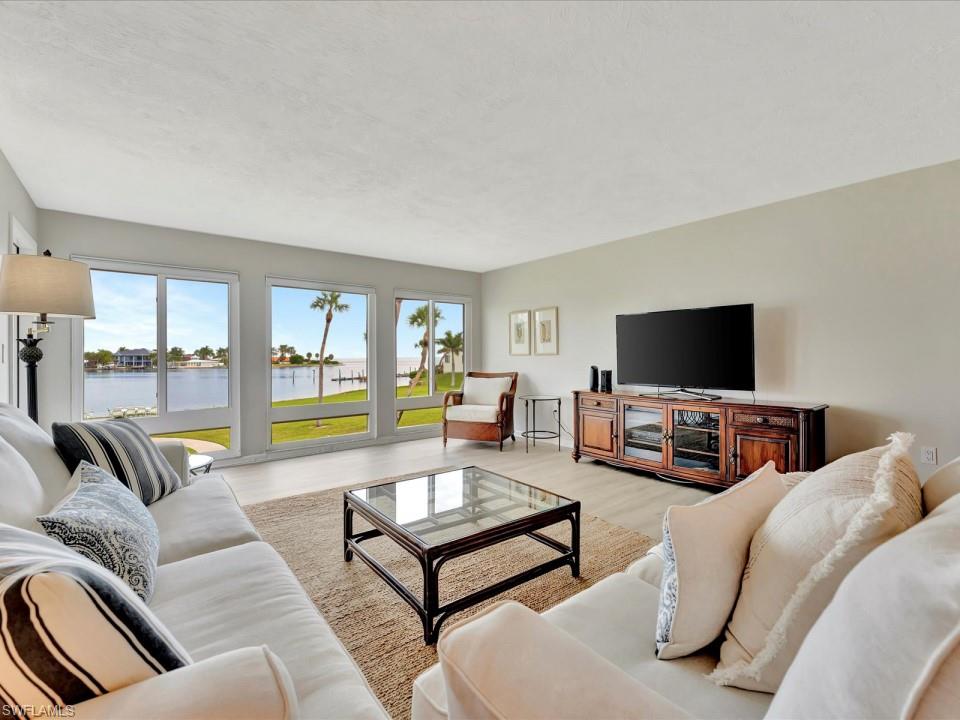The image showcases a spacious, elegantly decorated living room with large windows overlooking a serene waterway that opens up to what appears to be the ocean, framed by lush green grass and palm trees. Inside, the room features off-white or cream-colored walls, a white ceiling, and light wood flooring. The seating arrangement includes a beige or off-white sofa and loveseat, both adorned with an array of throw pillows, including navy and white striped, solid off-white, and blue and white patterned ones.

In the middle of the seating area sits a dark rattan-colored coffee table with a glass top, placed on a large beige rug. To the back of the room, there's a brown wooden chair with white cushions, accompanied by a small side table and two pictures hanging above it. Adjacent to this setup, a sleek entertainment center made of natural wood with glass doors hosts a large flat-screen TV and is flanked by speakers and additional black accents. The room's overall aesthetic is light and airy, with a color palette of neutrals complemented by splashes of navy blue and black, perfectly harmonizing with the breathtaking outdoor view.